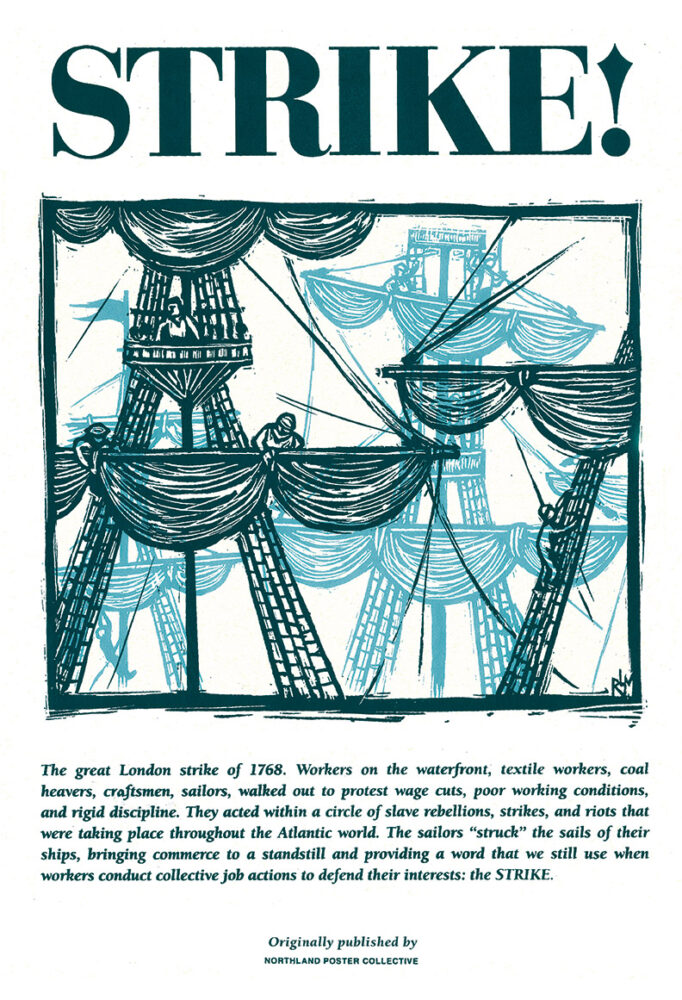This illustration depicts "The Great London Strike of 1768" and features prominently bold, dark blue letters at the top, exclaiming "STRIKE!" On the poster, workers are seen furling the sails on ancient ships reminiscent of pirate vessels, capturing a moment when sailors, craftsmen, textile workers, coal heavers, and waterfront workers walked out to protest wage cuts, poor working conditions, and rigid discipline. A man can be seen climbing the ropes up to the sails, another person is positioned in the crow’s nest, and several individuals are folding sails. The protest was part of a larger wave of strikes, slave rebellions, and riots across the Atlantic world, effectively bringing commerce to a standstill. This action gave rise to the term "strike" as it is used today. The hand-drawn illustration, likely screen-printed with a layered dark blue and light blue color scheme, is detailed with black outlines creating a strong visual contrast. At the bottom, it notes that the piece was originally published by the Northland Poster Collective.